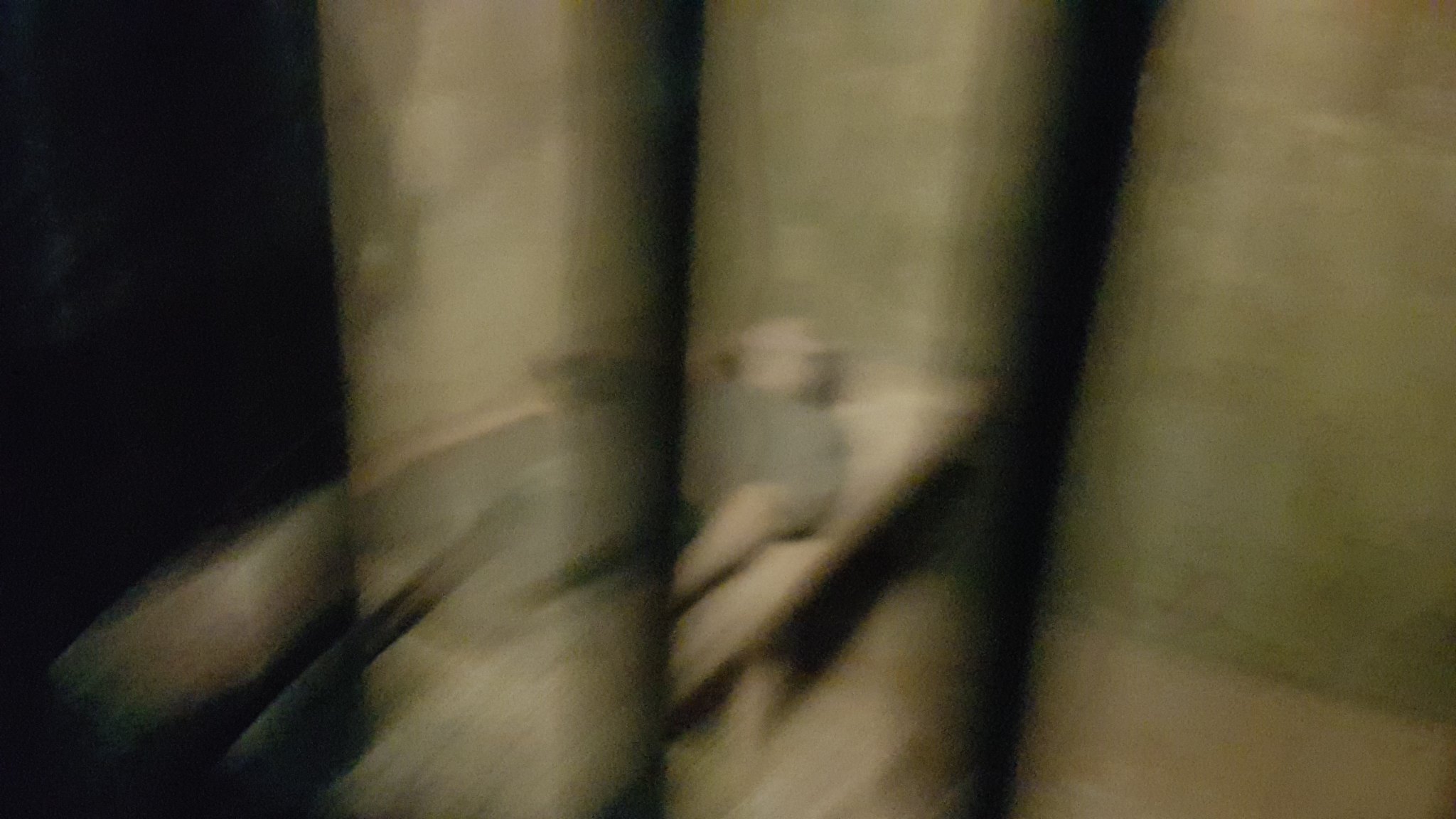In this somber and obscured image, the composition is dominated by a dull, grayish hue that lends an air of bleakness. Despite the overall vagueness and blurriness, upon closer examination, a lone figure becomes discernible. This person is reclining on what appears to be a rudimentary wooden plank, positioned within the confines of a stark cell. The individual's head is nestled into the corner of the room, and they are clad in gray fabric that blends with the muted tones of the setting. The scene is framed by the bars of the cell door, which is partially swung open, hinting at the presence of an unseen figure beyond the frame. The overall atmosphere is one of isolation and desolation, captured through the austere and minimalistic depiction.